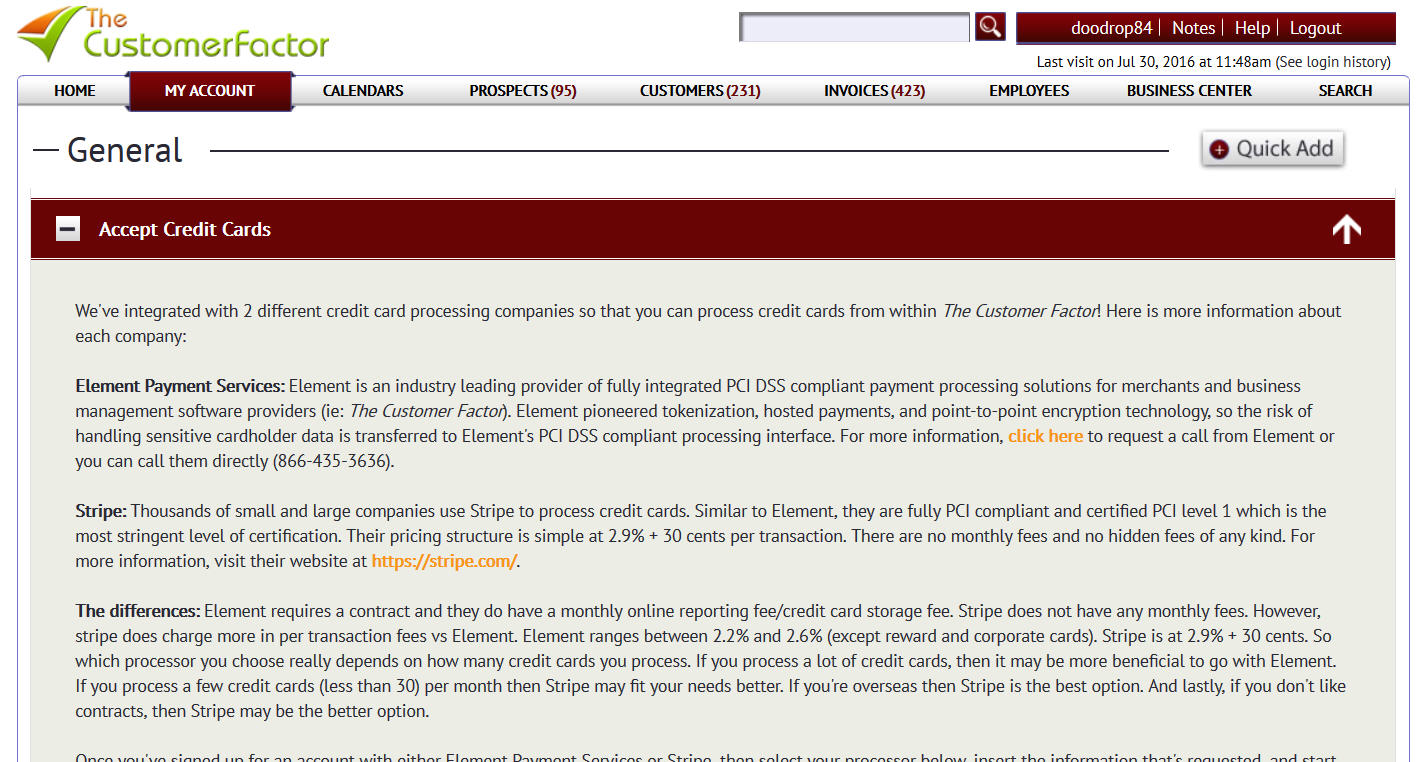The web page displayed is from a company called "The Customer Factor." In the upper left-hand corner, the company name is prominently featured with "The" in orange and "Customer Factor" in avocado green. To the left of the name is the company's logo—a triangular shape combining red and green sections. To the right of the logo, there is a search box. Further to the right, displayed in white text on a dark brown ribbon, are the username "DoDrop84," followed by options labeled "Notes," "Help," and "Logout."

Beneath this ribbon, in small black text, is the information: "Last Visit on July 30, 2016, at 11:48 a.m." with a parenthesis containing "See Login History." Below this, the main page features a silver banner with several navigation options from left to right: "Home," "My Account," "Calendars," "Prospects (95)," "Customers (231)," "Invoices (423)," "Employees," "Business Center," and "Search." In this context, "My Account" is highlighted in chocolate brown with white text.

The section below begins with the word "General" in black text, followed by a line that stretches across the page to a button labeled "Quick Add." This button is gray with "Quick Add" in black text and features a chocolate brown circle with a white plus sign inside it.

Directly below, a chocolate brown banner spans the width of the page with the words "Accept Credit Cards" in white text. Adjacent to this banner, a silver box contains a minus sign, and at the far right, there's an upward arrow in white. The rest of the page has small black text on a silver-gray background. The topmost sentence reads: "We've integrated with two different credit card processing companies so that you can process credit cards from within The Customer Factor!" 

The page provides detailed information about two credit card processing companies, Element Payment Services and Stripe, each described in a dedicated paragraph. Following these, a section titled "The Differences" compares the two options, although the comparison and subsequent text are cut off in the image.